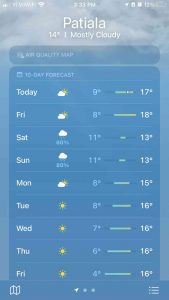This is an image of a weather forecast page for Patiala. The forecast spans approximately 10 days. The top-left corner of the image is quite blurry, making it difficult to discern the exact time, possibly 8:33. Below the time, there is a label indicating "air quality map." At the top of the page, the current temperature is displayed as 14 degrees Celsius with a "mostly cloudy" condition. 

Today's low is 9 degrees, with a high of 17 degrees expected. The forecast for the following days includes:
- Friday: mostly cloudy.
- Saturday: a 40% chance of rain.
- Sunday: an 80% chance of rain.
- Monday: probably cloudy with temperatures ranging from 8 to 15 degrees.
- Tuesday, Wednesday, Thursday, and Friday: sunny conditions, with temperatures around 8, 7, 6, and 4 degrees respectively for the lows, and 15 and 16 degrees for the highs.

At the very bottom of the image, there is an overall weather summary, but the text is difficult to read due to the image's blurriness. Overall, the image is fairly unclear, making it challenging to decipher specific details.